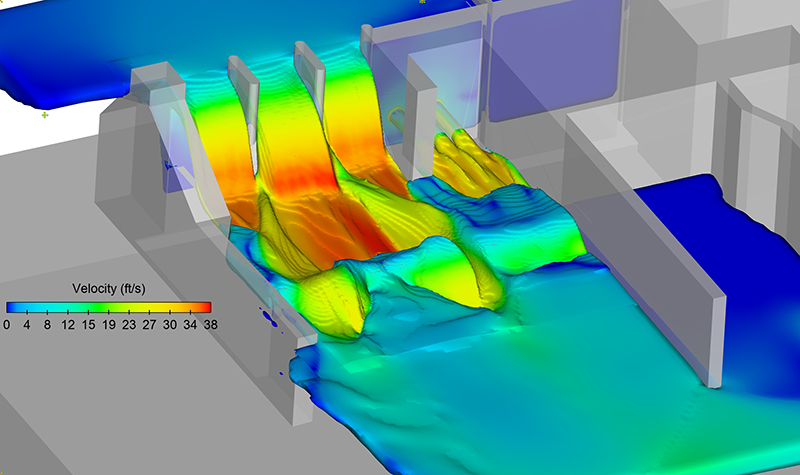This detailed 3D computer model visually represents a dam, showcasing the dynamic flow of water through three primary channels, each descending into a basin below. The depiction emphasizes a man-made structure designed to guide water from an upper body through these divided waterways, creating a cascading waterfall. The entire scene is framed by a transparent, gray framework that highlights its computer-generated nature. The water's velocity is vividly illustrated using a color-coded thermal key, ranging from zero to 38 miles per hour, located centrally within the model. The velocity colors transition through a spectrum from dark blue, indicating lower speeds, to red for the highest velocities, providing a clear visual understanding of flow dynamics. A legend to the side correlates these colors with their respective speeds in feet per second, enhancing the educational value of the model.